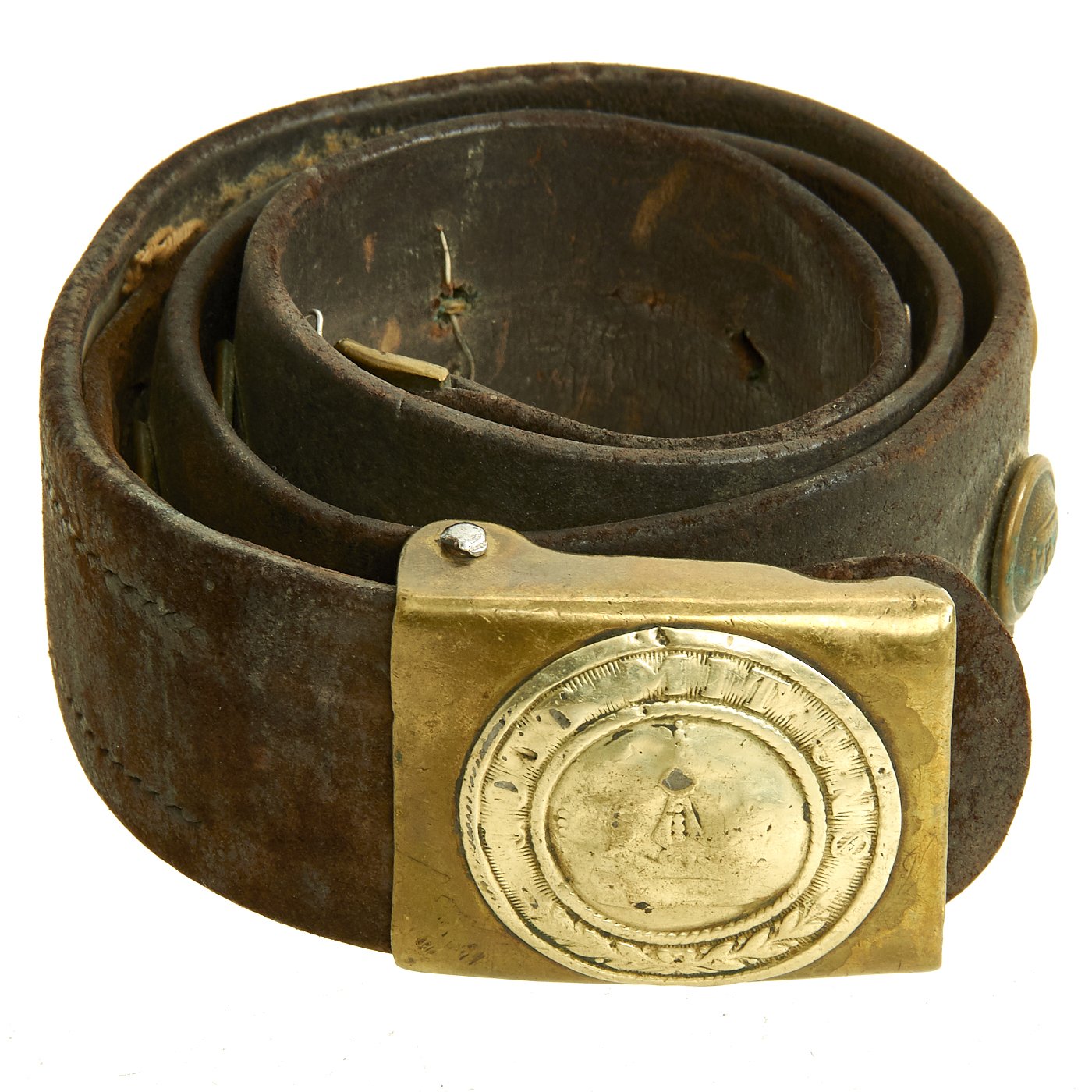This photograph captures a close-up image of a very old leather belt coiled together, set against a solid white background reminiscent of a museum archive. The belt itself is predominantly brown, although it appears darker and almost black in certain areas due to its age and extensive wear. The leather shows significant signs of deterioration, with noticeable cracks and extreme wear around the belt holes. Running along the middle of the belt is visible stitching, further emphasizing its craftsmanship.

The focal point of the image is the gold belt buckle, which is rectangular with intricate details that have eroded over time. At its center, there is a lighter gold circular coin that appears to have once held distinct engravings. Despite the wear making it challenging to discern, a few letters "MIT" and "UNS" can be identified, along with some leaf motifs engraved at the bottom. This coin adds a historic and artistic touch to the otherwise utilitarian object, hinting at a storied past.